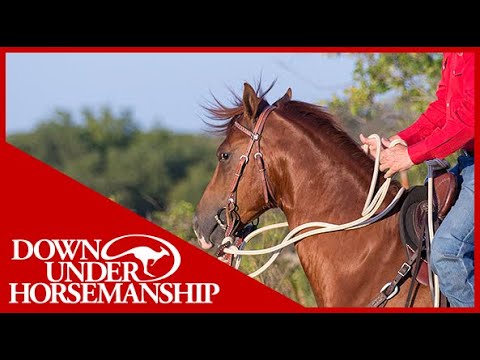The image features a brown horse viewed from the side, with a rider wearing a red shirt and blue jeans, whose head is cut off from the frame. The rider, with light skin, holds a white rope tied to the horse's brown leather harness and sits on a dark brown saddle with matching leather straps. The horse’s shiny fur is prominently visible, and the background consists of blurry green trees and a bright blue sky, indicating a sunny outdoor setting. The image is framed with black borders at the top and bottom and a smaller red border inside. On the left side, a red background displays the white text "Down Under Horsemanship," accompanied by a small image of a kangaroo.